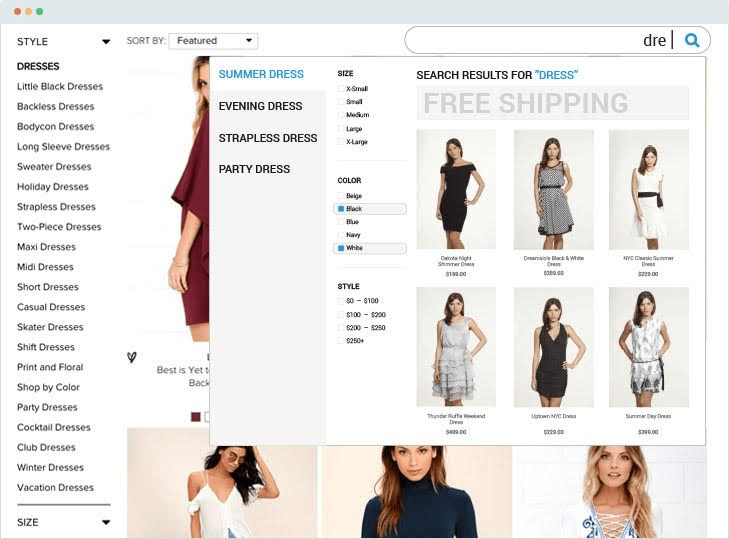The image depicts a detailed user interface of an online shopping platform. At the top, there's a grey navigation bar featuring several options, including a red, yellow, and green circle indicating different controls. Options such as 'Style,' 'Drop-down,' 'Insert,' 'Buy,' 'Feature,' and 'Move All' are visible. A section with a vertical blue line includes a magnifying glass icon for search functionalities and a list highlighting various dress categories such as: "Little Boy Dresses," "Breakfast Dresses," "Bodycon Dresses," "Long Sleeve Dresses," "Sweater Dresses," "Holiday Dresses," "Strapless Dresses," "Two-Piece Dresses," "Maxi Dresses," "Mini Dresses," "Short Dresses," "Casual Dresses," "Skater Dresses," "Shoes Dresses," "Parents in Floral," "Party Dresses," "Cocktail Dresses," "Club Dresses," "Winter Dresses," "Vacation Dresses," "Summer Dresses," "Evening Dresses," and "Party Dresses." Additionally, there's a size filter including options for sizes 1 through 5, Small, Medium, and Large.